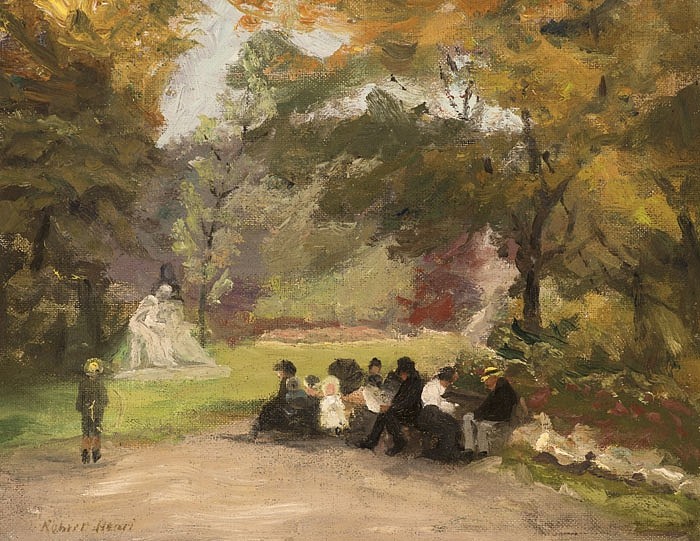In this vibrant watercolor painting, likely created by an artist with a name resembling "Krohrirhenri," an outdoor family gathering unfolds in an impressionistic style. The scene is set in a picturesque park during the fall season, characterized by an array of big green trees adorned with yellow, orange, and red leaves. The setting features a large dirt road bordered by rocks, where a cluster of about eight to ten people are seated at the edges, possibly enjoying each other's company and the serene environment. Off to the side, a small boy walks along the path, possibly holding a stick or a hula hoop, adding a sense of movement to the tranquil scene. In the background, a silver statue of a person stands, complementing the natural beauty with a touch of artistry. The overall ambiance conveys a peaceful daytime gathering, with detailed yet nondescript faces that emphasize the impressionistic nature of the artwork.